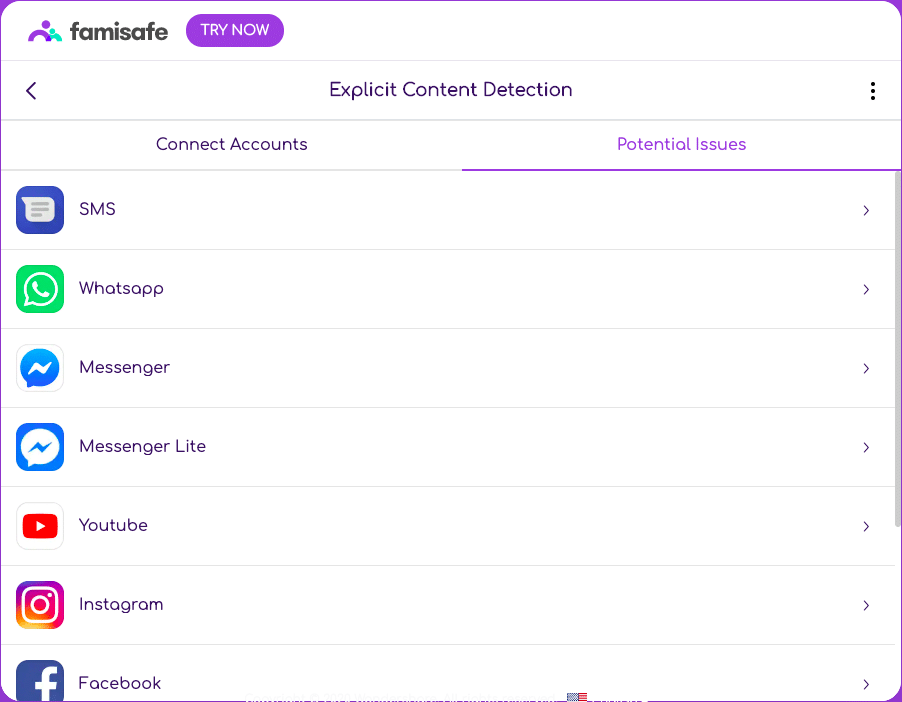The image displays a webpage titled "FAMISAFE" prominently in the top left corner, spelled out as F-A-M-I-S-A-F-E. Adjacent to this title, there is a purple button labeled "Try Now" in white text. Directly below, a banner reads "Explicit Content Detection," accompanied by a dropdown menu towards the right.

Below this banner, two tabs are visible: "Connect Accounts" and "Potential Issues," with the latter highlighted in purple and underlined. The left-hand side of the webpage lists several apps, each indicated by their respective icons:

1. SMS – With an icon aligned to the left and depicted by its logo.
2. WhatsApp – Also displayed with its recognizable icon.
3. Messenger (Facebook Messenger) – Denoted by its logo.
4. Messenger Lite (Facebook Messenger Lite) – Identified by the Messenger Lite logo.
5. YouTube – Marked with its familiar icon.
6. Instagram – Represented by the Instagram logo.
7. Facebook – Shown with the Facebook icon.

Each app entry has a right-facing triangle at the end of its respective line, indicating further options or details.